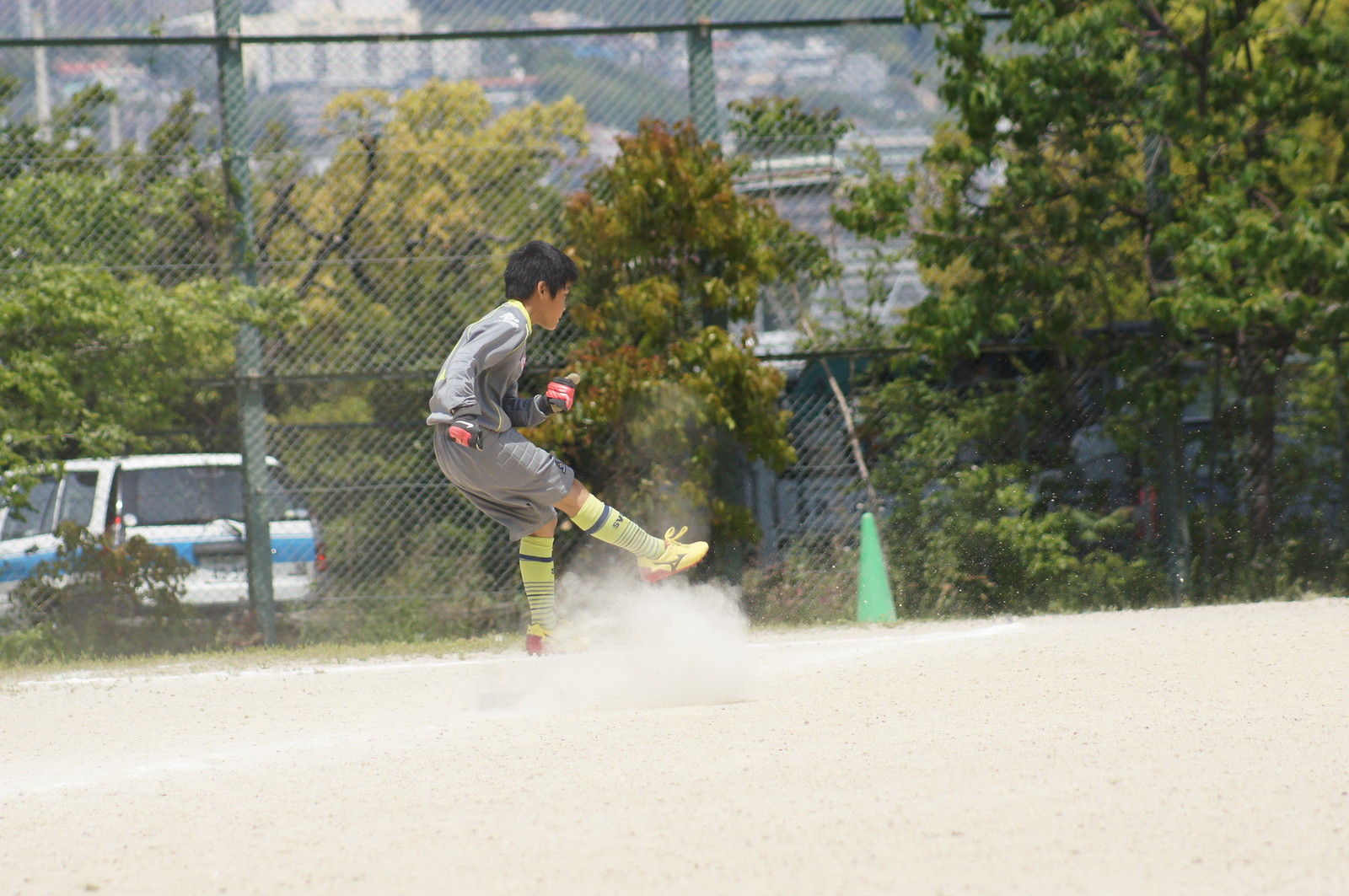In this photograph, a young boy, likely of Asian or Hispanic descent, is captured in the midst of a playful kick on a dusty baseball field, hinting at a soccer game despite the lack of a visible ball. His skin is dark, and he has dark hair. Dressed in a gray uniform consisting of a shirt and shorts, he stands out with his bright yellow cleats, which feature red heels, and knee-high yellow socks adorned with black stripes. The boy also wears black and red gloves, possibly indicating his role as a goalie on his team. Surrounding him is a plume of dust at his feet, suggesting the intensity of his recent kick. A green cone sits approximately three feet from him, adding a touch of color to the dirt-covered scene. Beyond the fenced perimeter of the field, a white and blue striped vehicle is parked, and the backdrop features green shrubbery and trees, with blurred buildings perched on a distant hill, indicating a cityscape. The setting appears to be during the middle of the day, under natural daylight. There is no text or date marking on the photograph.